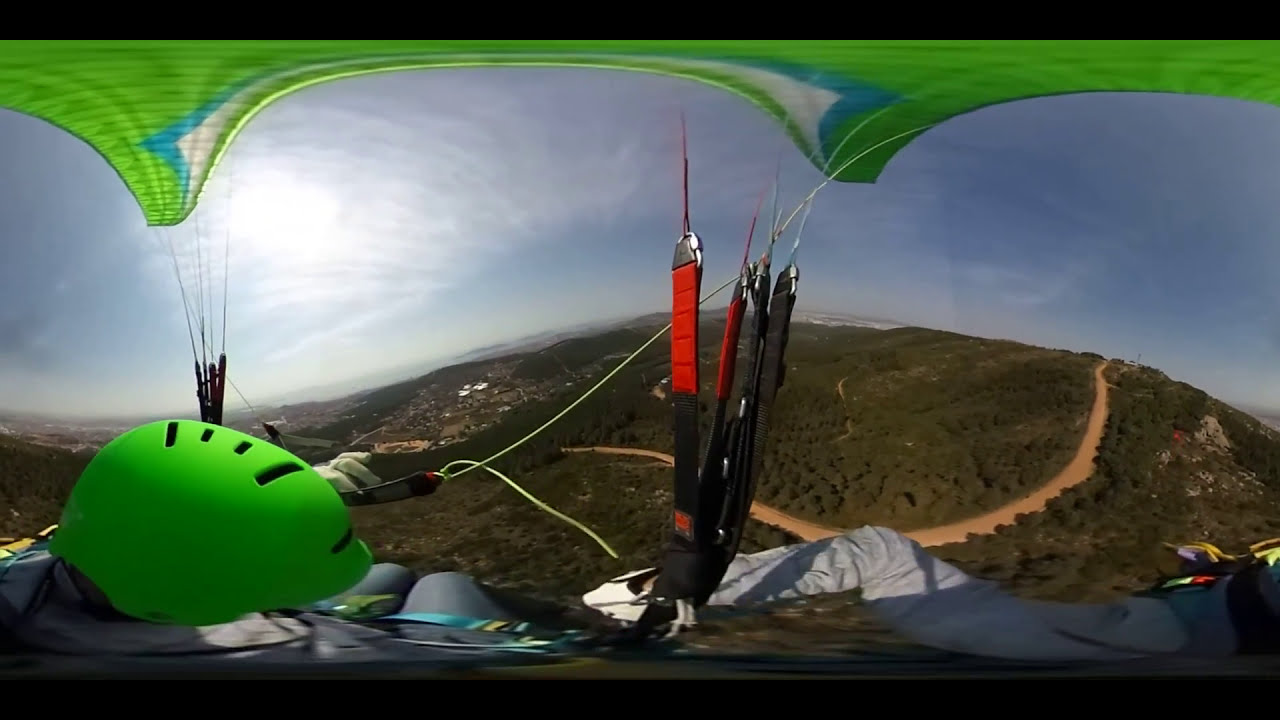This overhead photograph captures a vibrant scene from a hang glider, immersed in an adventure high above a landscape. Dominating the foreground is the pilot, distinguishable by a bright lime green helmet adorned with black stripes, positioned towards the bottom left of the image. The pilot's knees are tucked up near their chin, and they are gripping onto ropes or handles essential to the hang glider's navigation.

Suspended above the pilot is the glider canopy, which shares the helmet’s vivid lime green hue. The canopy has a distinctive design, featuring three sweeping arches that converge at specific points tied together by white strings. These strings connect to thicker black and red straps, providing both structure and support to the glider.

In the background stretches a scenic view of a hilly landscape. The hill's surface, a mix of dirty green and brown hues, is dissected by a tan trail winding across it. At the base of the hill, a roadway runs horizontal and is depicted in tones of gray and white. The expansive sky, transitioning from a bright blue on the left to a deeper shade on the right, creates a striking backdrop. On the far right of the horizon, houses and structures pepper the edge of the hill, adding depth and context to the scene.